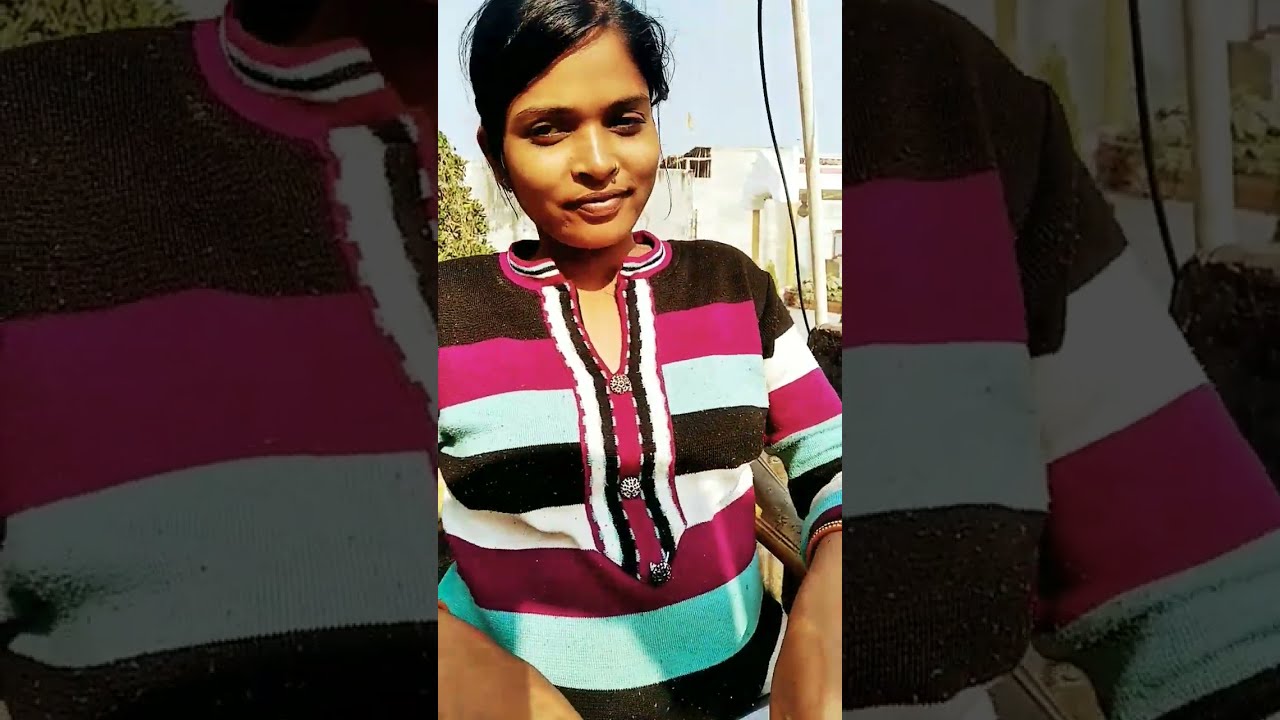The image showcases a young woman, possibly of Indian or Middle Eastern descent, smiling warmly at the camera. She is wearing a stylish sweater with vertically repeating medium to thick stripes in black, pink, and green, which extends just past her elbows and leaves her forearms bare. Her short black hair is neatly pulled back and parted on the left. The setting appears to be a city under a bright blue sky, with buildings and trees in the distant background, suggesting a pleasant sunny day. The photograph is presented in a landscaped format featuring a central portrait of the woman from her waist up, flanked by two smaller side panels that highlight fragments of her striped sweater against an opaque black background. Her relaxed posture, with arms bent in front of her, conveys a casual and comfortable demeanor, possibly enjoying a leisurely moment seated outdoors.